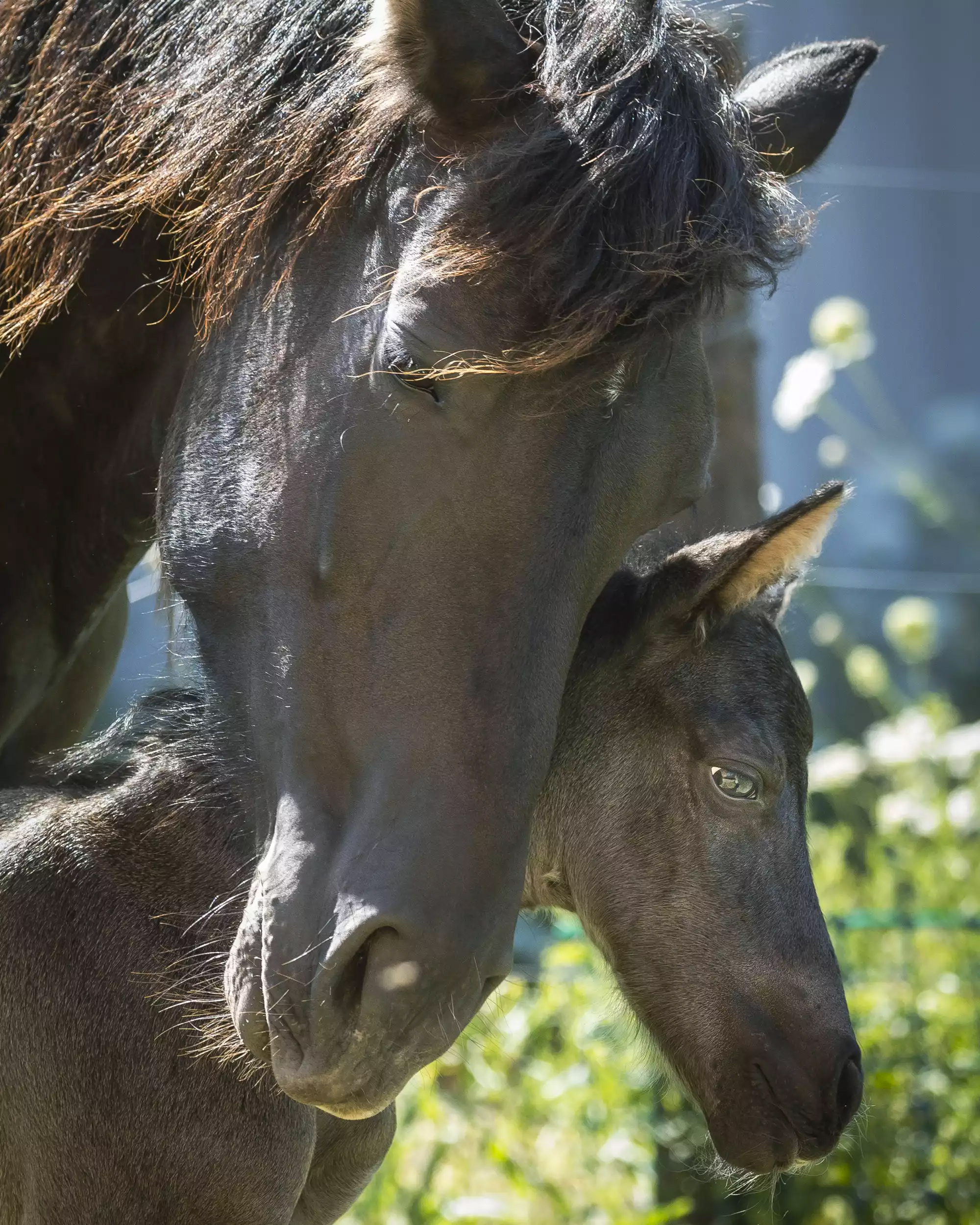In this captivating outdoor image, a dark-colored mare, possibly a super dark bay or black, tenderly nuzzles her foal, exhibiting a profound bonding moment. The mare, with her medium-length, slightly wavy mane that is tussled by the wind and subtly bleached brown, holds her head down, arching her neck in a protective gesture. She features a small white star on her forehead and appears nurturing, with a little hair visible on her face and ears. Beside her stands her foal, who mirrors her dark coloration and looks contented with its soft-looking nose and cute fuzzy ears. The foal's short fur and small fuzzy mane indicate its youthful age, and its eyes are striking, described as a grayish-greenish hue. The surroundings include dandelions, grass, and a fence, further enhancing the serene and natural setting depicted in the close-up shot. The image beautifully captures the essence of maternal care and the intimate connection between the mare and her foal, evoking a sense of tranquility and the timeless beauty of nature.